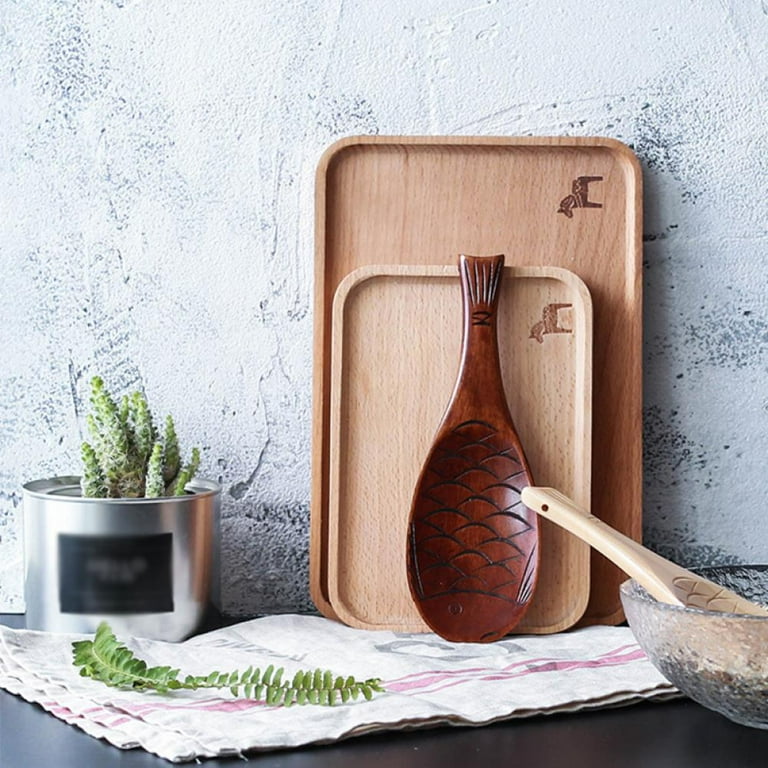In this photograph, a collection of wooden kitchen tools and decor items are arranged on a matte black dresser against a rough plaster wall with traces of gray peeking through. Central to the scene is a white towel with a red stripe, upon which lies a green fern frond. Leaning against the wall are two light blonde wooden platters featuring images of horses, alongside a platter shaped like a fish in darker wood. To the right, a frosted glass bowl holds another fish-shaped wooden spoon, matching the blonde wood of the horse platters. A stainless steel pot containing a succulent plant adds a touch of greenery to the left side of the arrangement. The image, set against what appears to be a rustic plaster or concrete wall, showcases an assortment of intricately designed kitchen tools and natural elements, blending practicality with aesthetic appeal.